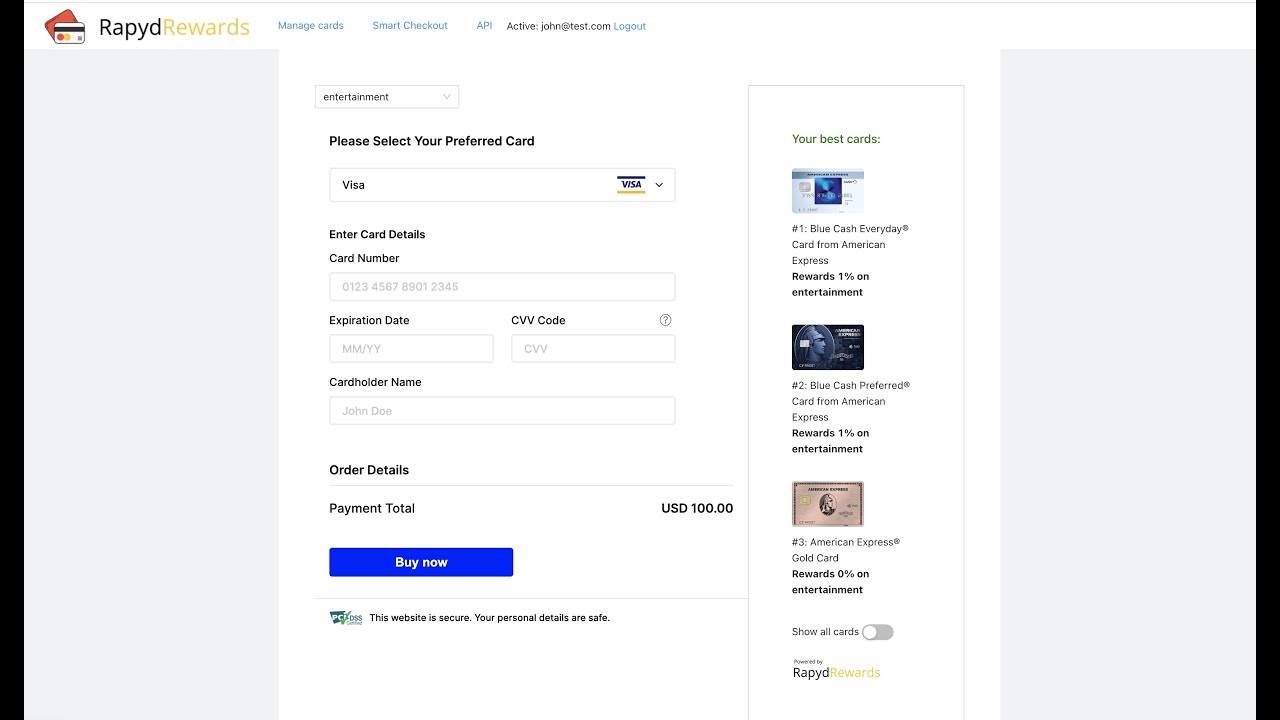The image displays a webpage for a payment interface titled "Rapid Rewards." At the top of the page, there are illustrations of a shopping cart, a MasterCard, and another credit card. Below these icons, in blue text, it reads "Manage Cards Smart Checkout API." Following this text, the page displays the account information "ActiveJohnAtTest.com" along with a "Logout" option also in blue.

Underneath this header, there is a drop-down box labeled "Entertainment." Next, it instructs the user to "Please Select Your Preferred Card," with another drop-down box below it. The default selection in this box is "Visa," accompanied by a blue and yellow Visa logo on the right-hand side.

Further down, the section titled "Enter Card Details" appears. It includes a long rectangular input box labeled "Card Number" with placeholder numbers indicating the required format. Beneath this input area, there are two adjacent rectangular boxes: one for the "Expiration Date" and the other for the "CVV Code," accompanied by a small circle with a question mark icon for additional information.

Following these fields, the form requests the "Card Holder Name" with another rectangular input box. 

The section "Order Details" is displayed next, summarizing the "Payment Total" as "USD $100." A prominent blue rectangular button labeled "Buy Now" is positioned below the total. At the bottom of the form, a security assurance message reads, "This website is secure. Your personal details are safe."